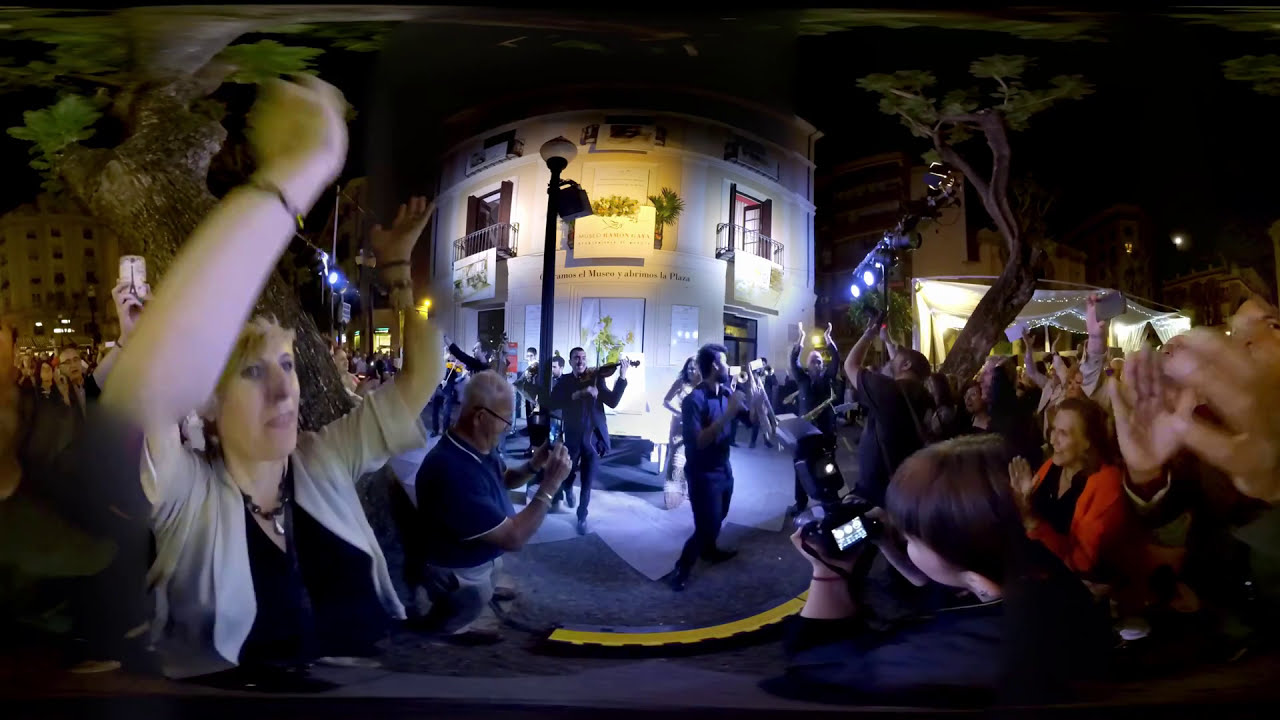In this photograph, there is a lively street celebration taking place at night, captured with a slightly distorted lens giving it a curved appearance. The scene is dominated by a group of people dancing, clapping, and generally reveling in the moment. In the immediate foreground on the left, a white woman with light hair is exuberantly raising her arms, showcasing a beige overshirt layered over a black top, accompanied by several bracelets and a necklace. Next to her, a small child is focused on a camera. On the right side, a woman in a red cardigan over a black shirt is energetically clapping her hands. 

At the center of the image, a man holding a microphone appears to be the source of the musical excitement, while behind him, another man plays a violin. The background reveals a large, arched white building with multiple stories and balcony spaces, illuminated by streetlights. The sky is dark, indicating nightfall, and the scene is framed by oddly-shaped, bent trees on both sides. The crowd and musicians are bathed in light, enhancing the festive and joyous atmosphere of this nighttime street performance.